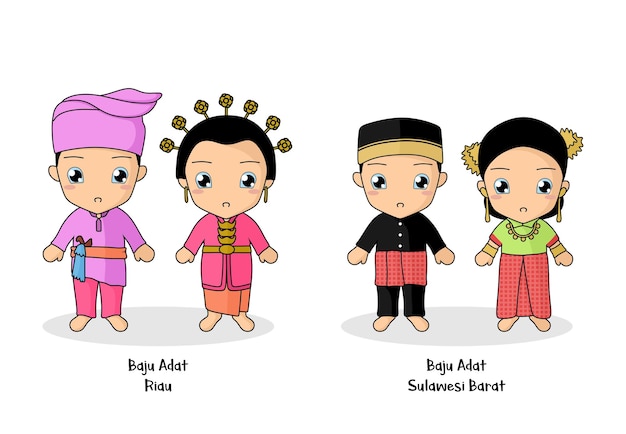This image features four anime-style characters standing on two gray ovals with no background or border. On the left gray oval, labeled "Baju Adat Riau," there is a boy and a girl. The boy is dressed in a purple karate-like outfit, which includes a purple hat, purple shirt, pink pants, and a belt with a blue tassel. The girl beside him has black hair adorned with pins and wears a pink jacket over an orange skirt, with a belt across her shirt featuring gold designs. On the right gray oval, labeled "Baju Adat Sulawesi Barat," another boy and girl are depicted. The boy wears a black and gold hat and a matching black and pink outfit. The girl standing next to him has black hair decorated with gold bows or jewelry and gold earrings. She is dressed in a skirt that matches the red part of the boy’s shirt and wears a neon green shirt with red stripes and a necklace.